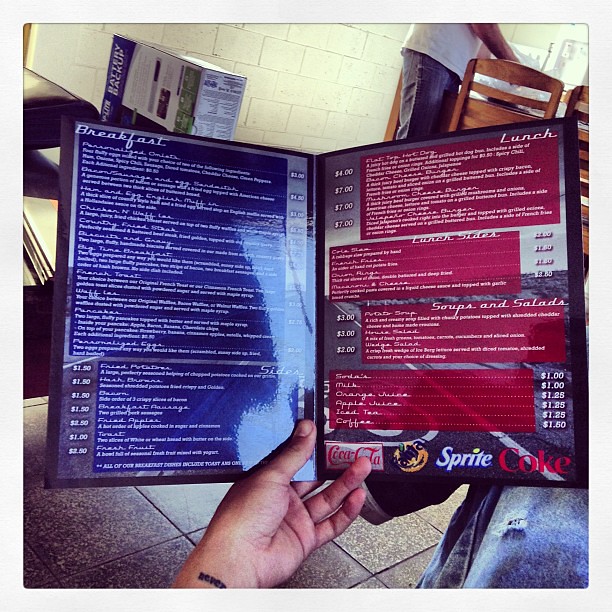In the image, there is a close-up partial view of an individual wearing jeans, focusing on their leg and hand. The hand, adorned with a black ink tattoo on the wrist, is holding a bi-fold menu. On the left side of the menu is the breakfast section, featuring a list of breakfast items against a blue background, with the text displayed in white ink. On the right side, the menu lists lunch options, highlighted in red with white text. Additionally, the top of the lunch section features logos of popular beverage brands: Coca-Cola, Fanta, Sprite, and Coke. The composition provides a detailed glimpse into the menu offerings and the person holding it.